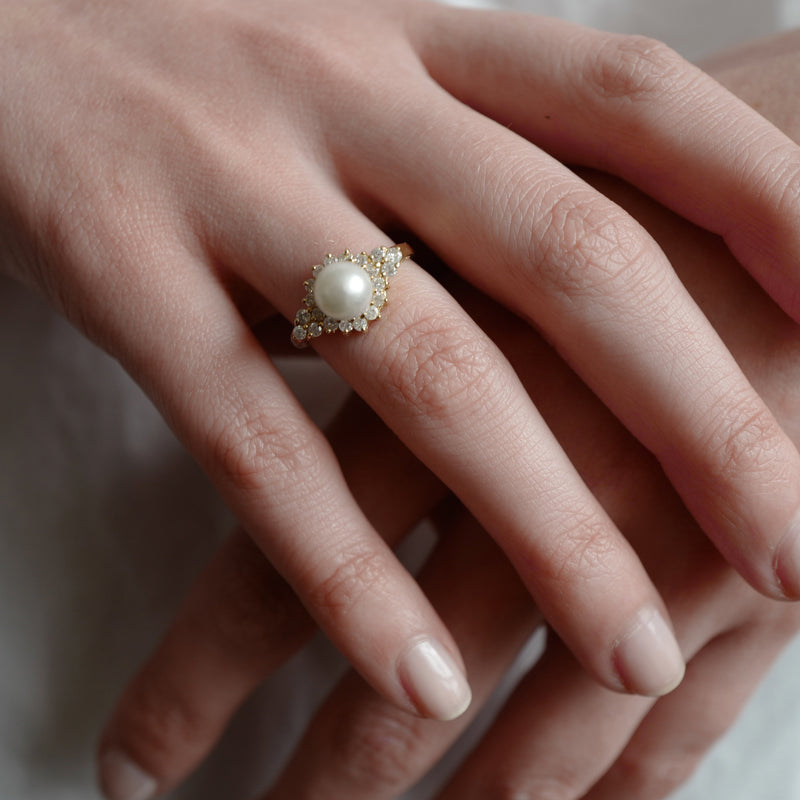This image is a professional and detailed wedding photograph focusing on the bride's hands, which are elegantly posed to showcase her exquisite pearl engagement or wedding ring. The bride's right hand, adorned with the ring, rests gracefully atop her left hand, casting delicate shadows that enhance the photo's realism. She has small, fair-skinned fingers, free of any tanning or imperfections, and her natural nails are neatly trimmed and painted with a subtle beige polish, without any fake enhancements.

The ring itself is a stunning piece of jewelry, featuring a lustrous white pearl set in the center of a diamond-shaped arrangement composed of numerous small diamonds, all mounted on a gold band with intricate gold and white accents. The background is a pristine white velvet cloth or possibly a white garment, further emphasizing the purity and elegance of the moment. This meticulously edited photograph captures the essence of the bride's beauty and the significance of the occasion.